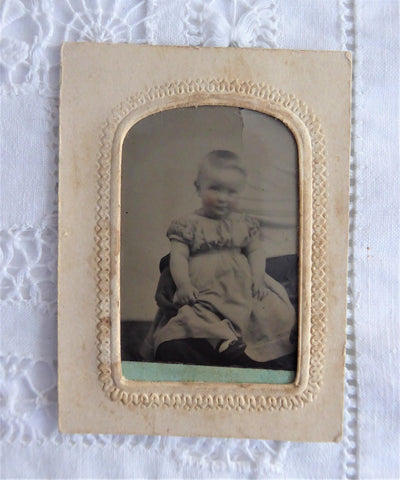This image captures a vintage black-and-white photograph of a young child, possibly around one year old, seated and gazing thoughtfully into the camera. The child’s attire—a long dress with an empire waist and puffy sleeves—suggests a time period between 50 and 100 years ago, and the short hair and patent leather shoes add to the old-time appeal. The photograph, slightly blurry and of low quality, is framed with a worn, beige papery border showing signs of age. It rests on a white tablecloth or doily with intricate crocheted trim, evoking a sense of nostalgia. This timeless image, likely taken in the 1960s or earlier, provides a glimpse into the past, featuring a chubby-cheeked child whose gaze captivates and holds a piece of history within its frame.